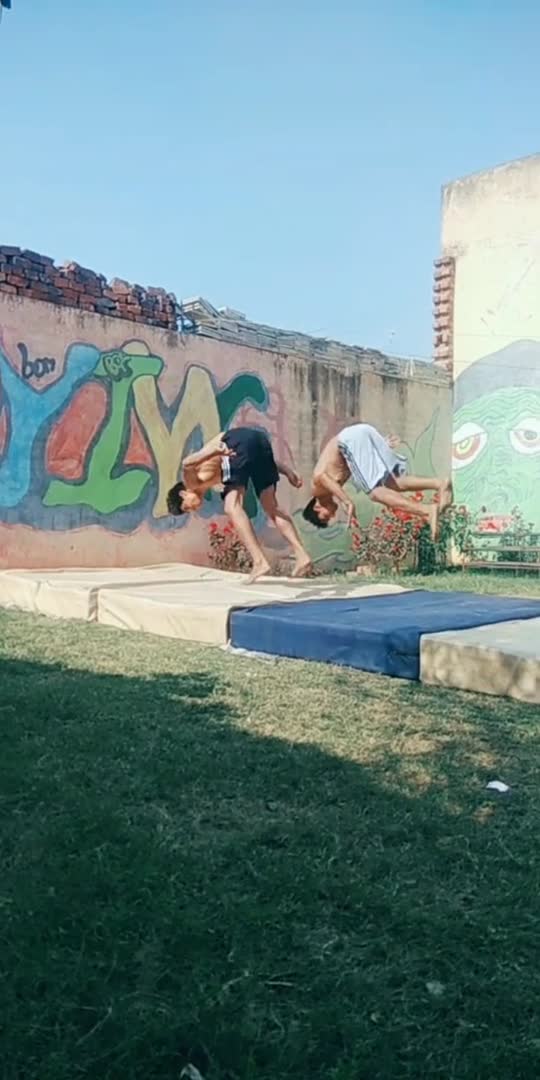The image captures a dynamic outdoor scene featuring two shirtless young boys in mid-air, perfectly synchronized in their front flips. They are leaping over a series of gymnastics mats arranged horizontally on a grassy lawn. The mats consist of alternating dull yellow and blue colors. The backdrop consists of a soft pink concrete wall adorned with vibrant graffiti that spells out "YIN" in a mix of blue, green, and yellow letters against a reddish background. To the right, another taller yellow wall is visible, sporting graffiti that resembles either a frog or a lizard's face. The bright blue sky and the shadows cast by trees further frame this energetic and adventurous moment of play and skill.